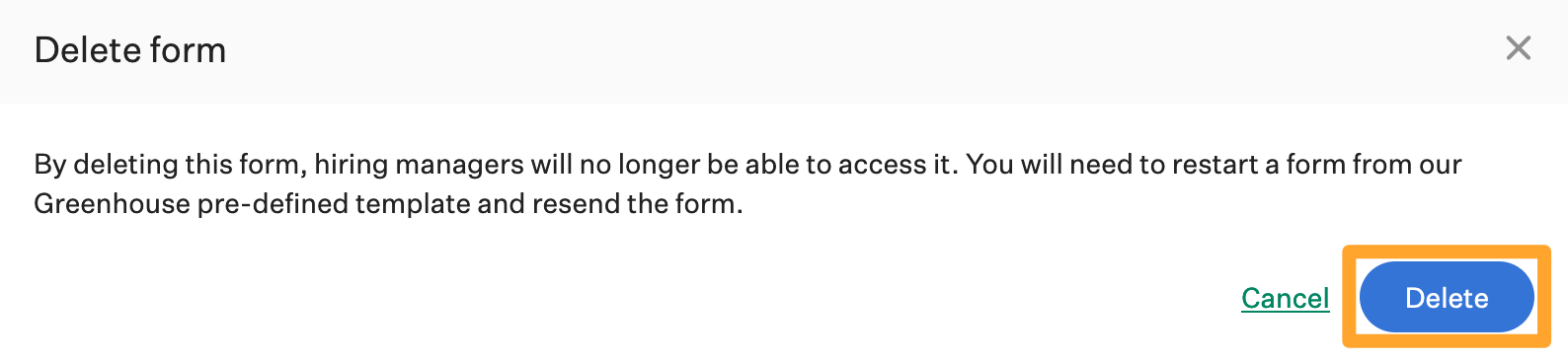In this image set against a solid white background, black text dominates the upper section. In the upper left corner, the text reads "Delete Form." On the opposite side, in the upper right corner, there is a gray 'X' icon. Below this header, a cautionary message is displayed twice, stating: "By deleting this form, hiring managers will no longer be able to access it. You will need to restart a form from our Greenhouse predefined template and resend the form." 

Further down, aligned to the right, green underlined text provides the option to "Cancel," followed by an orange box containing blue text that reads "Delete." This arrangement indicates an interface designed to confirm the deletion of a form, ensuring users are aware of the consequences and providing them with options to either proceed or cancel the action.